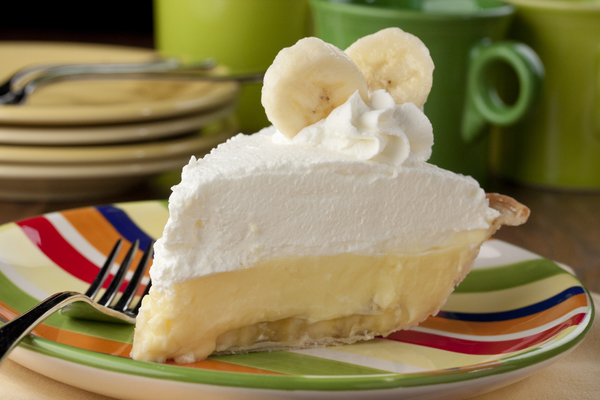An artfully positioned slice of banana cream pie is showcased on a vividly striped plate adorned with white, green, beige, blue, orange, red, and yellow hues. The delectable dessert features a base layer of bananas, a layer of creamy custard, and a generous topping of white whipped cream, garnished with two slices of fresh banana. A fork rests invitingly next to the pie. Positioned on a bamboo-colored table, the scene also includes a green coffee cup and a stack of cream-colored plates with utensils in the blurred background. The colorful plate and the fresh, appetizing pie slice are the primary focus, highlighting the enticing presentation likely intended to promote the dessert.